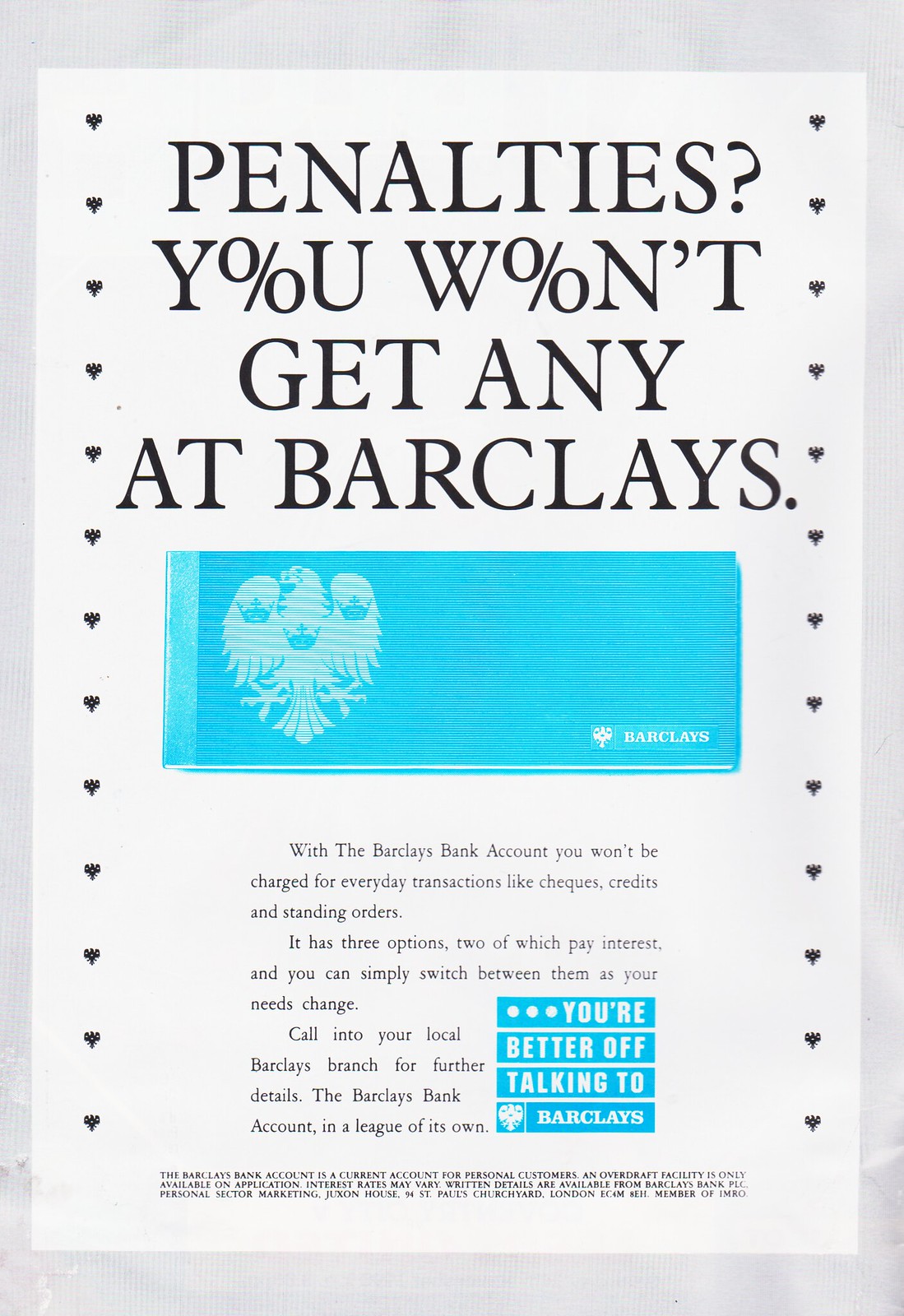This advertisement for Barclays Bank, featured in a magazine or newspaper, emphasizes their policy on avoiding penalties. The prominent headline reads, "PENALTIES?" followed by "YOU W%N'T GET ANY AT BARCLAYS," with the 'O's replaced by percentage signs for emphasis. Below this, a bright blue rectangle displays the Barclays logo and a stylized eagle with three crowns. The descriptive text below states that with a Barclays bank account, customers won't be charged for everyday transactions, including checks, credits, and standing orders. The ad highlights three account options, two of which offer interest, allowing customers to switch based on their needs. Additionally, it encourages potential clients to visit their local Barclays branch for more details, claiming the Barclays bank account is "in a league of its own." The right side of the ad features the phrase "You're better off talking to Barclays," with some finer print at the bottom that's difficult to read due to resolution. The ad's background is white, with the text and logos making a clear contrast against it.